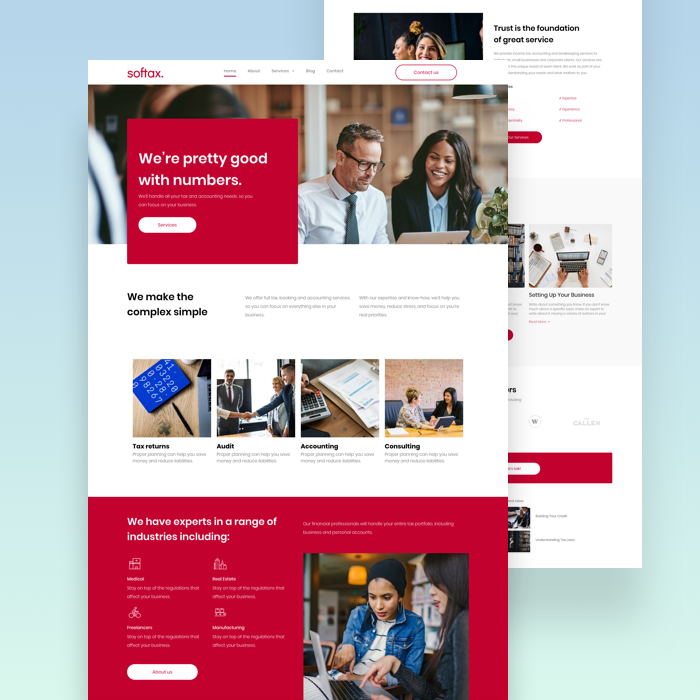The emergency webpage of Softax prominently features categories labeled Home, About, Services, Blog, and Contact. The company emphasizes the slogan, "Trust is the foundation of a great service," underscoring their commitment to reliable solutions. Softax prides itself on their numerical expertise, ensuring meticulous handling of all tax and accounting needs, allowing clients to focus on their business operations. Their services are designed to simplify complexity, encompassing tax returns, audits, accounting, and consulting. Softax boasts a team of experts proficient in diverse industries such as medical, professional services, and manufacturing. The color scheme of this image includes shades of blue, red, white, and black, creating a professional and trustworthy visual appeal.